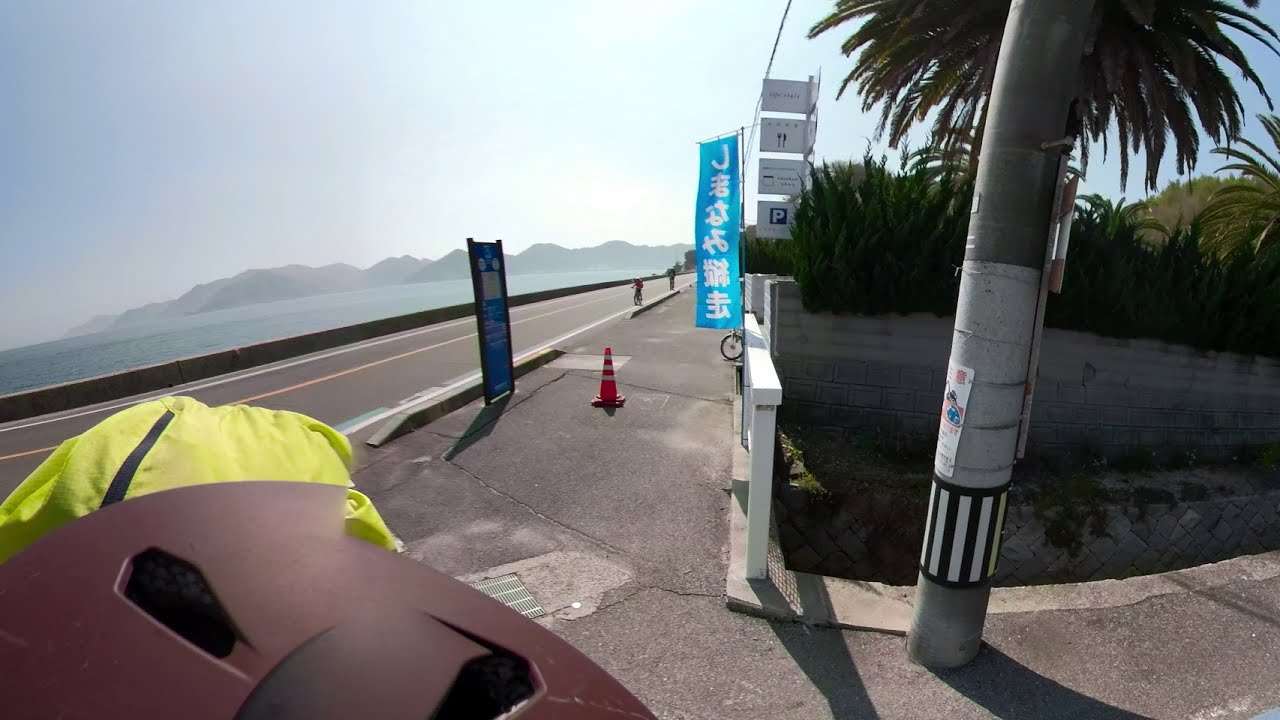This vibrant GoPro-type image, possibly a screen grab from a video, captures an outdoor street corner scene on a bright and sunny day. The viewer's perspective seems to be from a helmet cam, likely atop a motorcycle or scooter, suggested by the brown plastic object with yellow fabric at the bottom left, which appears to be the seat. The street corner is right across a narrow, two-lane highway marked by a yellow dividing line. This highway is walled off and seems to disappear over a cliffside, leading to a stunning view of the ocean. Beyond the ocean, you can see land rising into mountains, forming a picturesque inlet.

The sidewalk on the right side turns to go down another direction, featuring a tall metal pole, probably for a streetlight or stoplight, with a blue sign that includes what looks like Chinese or Japanese script. There is also a safety cone visible in the middle of the sidewalk. Adjacent to the sidewalk is a gray stone wall with green vegetation and some palm trees behind it, adding to the tropical ambiance.

In the upper left part of the image, the sky is mostly clear, flecked with bright white clouds, enhancing the overall brightness of the day. This comprehensive scene embodies the essence of a coastal street corner, blending urban elements with natural beauty.